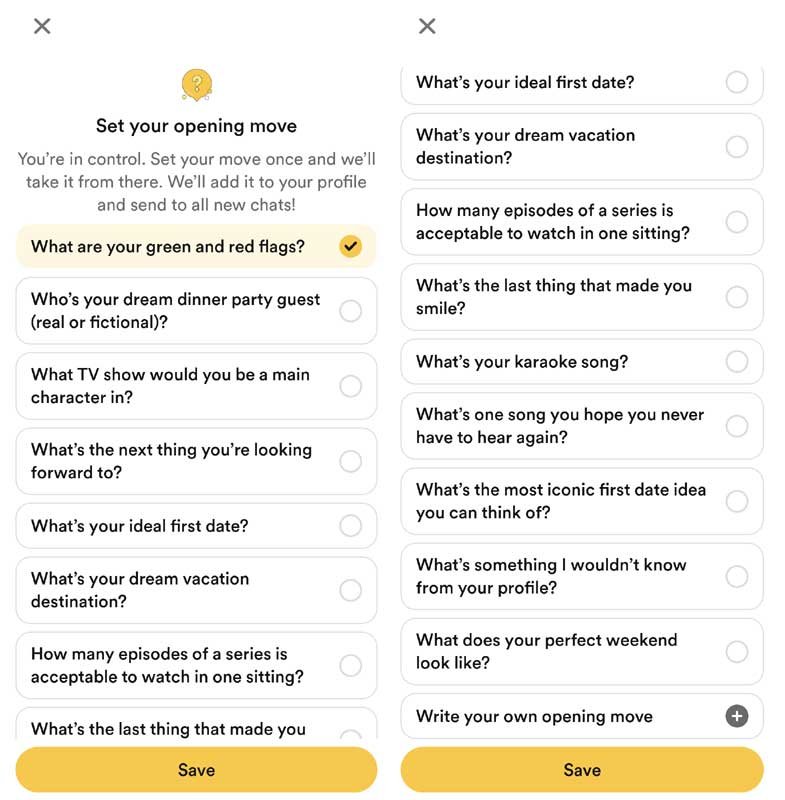The image is divided into two vertically rectangular frames, each showcasing screenshots from a cell phone app. Both frames prominently feature a close button (X) at the upper left. The left screenshot invites the user to "set your opening move" with the message: "You're in control. Set your move once and we'll take it from there. We'll add it to your profile and send it to all new chats."

Beneath this, several rectangular selection bubbles are listed with various questions, including:
- "What are your green and red flags?" (this option is checked)
- "Who's your dream dinner party guest, real or fictional?"
- "What TV show would you be a main character in?"
- "What's the next thing you're looking forward to?"
- "What's your ideal first date?"
- "What's your dream vacation destination?"
- "How many episodes of a series is acceptable to watch in one sitting?"
- "What's the last thing that made you," (incomplete phrase)

A yellow "Save" button is located underneath these options.

The right screenshot mirrors the left, showing partial duplicate content from the options:
- "What's your ideal first date?"
- "What's your dream vacation destination?"
- "How many episodes of a series is acceptable to watch in one sitting?"
- "What's the last thing that made you smile?"
- "What's your karaoke song?"
- "What's one song you hope you never have to hear again?"
- "What's the most iconic first date idea you can think of?"
- "What's something I wouldn't know from your profile?"
- "What does your perfect weekend look like?"
- "Write your own opening move"

This screenshot also concludes with a "Save" button. The app interface appears to be designed for personalizing user profiles with varied, engaging prompts to spark conversation in new chats.